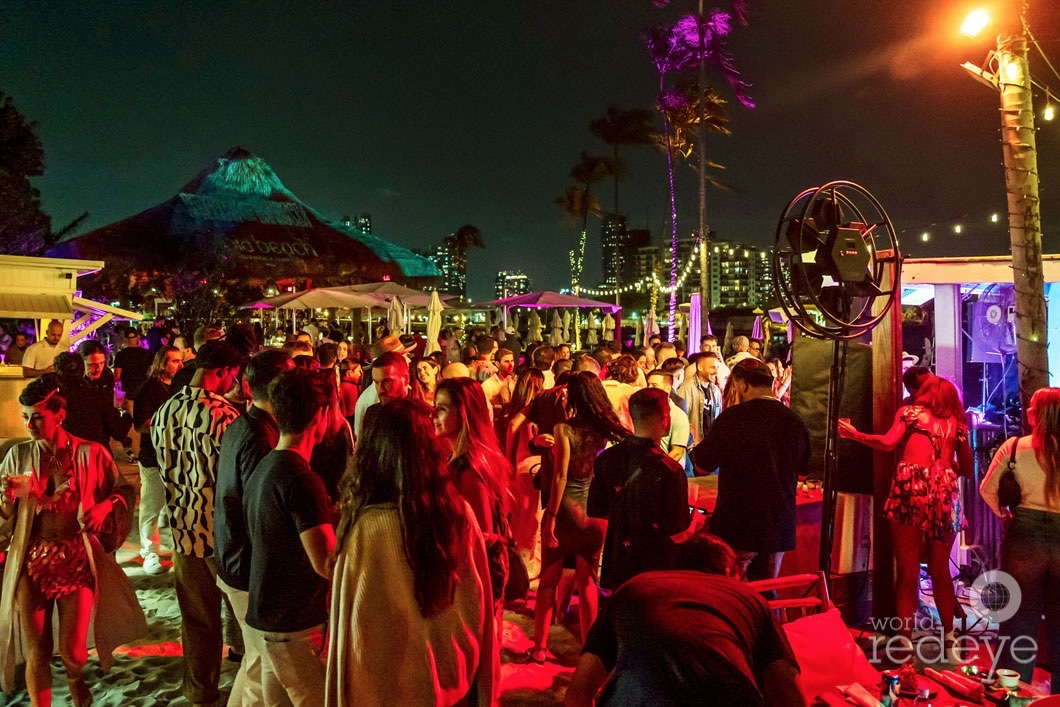The photograph depicts a lively nighttime carnival or party set in a warm climate, illuminated by red and white lights that cast vibrant hues across the scene. The sky is a deep black, dotted with scattered buildings and skyscrapers glowing with light, and a row of swaying palm trees adds to the festive atmosphere. A mountain resembling Mount Fuji is visible on the horizon, though the location remains ambiguous. The foreground is bustling with people dressed in summer attire, such as dresses, t-shirts, and shorts, engaging in dancing, talking, and drinking. Various shacks, tents, and what appears to be a shop can be seen, along with a standing fan or heater. Off to the left, there's a building with a triangular roof, and in the bottom right corner, there's a watermark reading "World Red Eye."